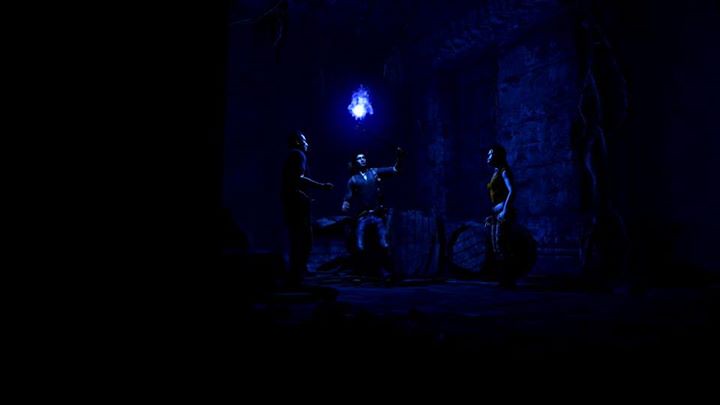In this atmospheric image, likely sourced from a video game or movie, a dim bluish light provides the sole illumination in an otherwise dark space. The light comes from a glowing orb hanging from the ceiling, partially covered by some material. The scene features three figures, their features barely discernible in the low light. One figure shows the side of their face, subtly lit. Another man, clad in a dark blue suit that blends into the shadowy surroundings, has his face, part of his chest, and a hand illuminated. The third figure, a woman in a reddish dress, is seen looking upward, with the side of her face and one bare arm catching the faint light's reflection. The trio appears to be either seated or standing around a circular opening in the stone floor of the building, further adding to the mysterious ambiance.